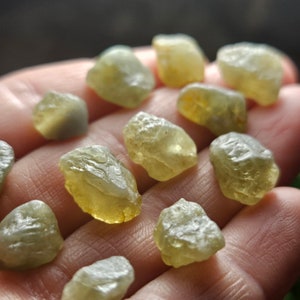The image is a close-up, slightly blurry shot of a hand held palm up, prominently displaying twelve small pebbles spread between the fingers. The background is a dark grey, adding emphasis to the hand and pebbles. The pebbles, nestled among the person’s four visible fingers, range in shape from round to elongated but share a predominantly circular form. These pebbles are light yellowish-olive to brown in color, with some of them exhibiting translucent parts while others appear solid, suggesting they might have originated from the same larger rock. The positioning shows four pebbles between the first two fingers, five between the second and third fingers, and three between the third and fourth fingers.